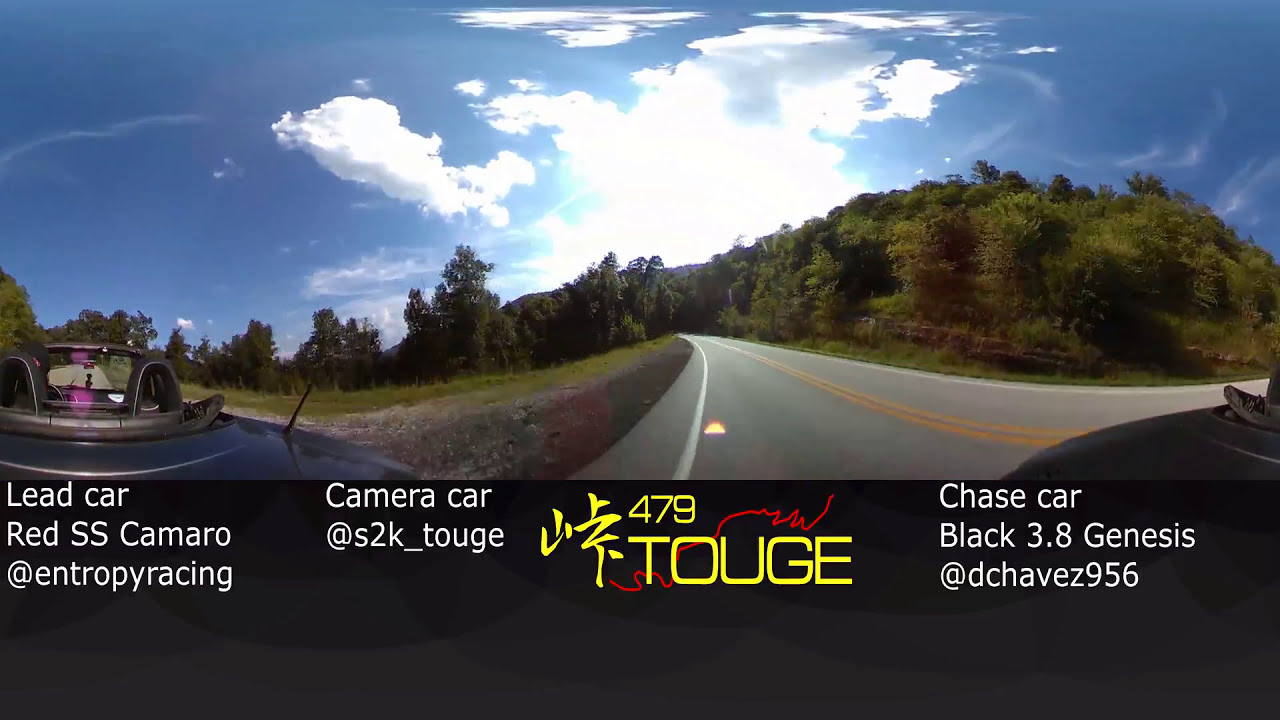A panoramic color photograph captures a landscape scene dominated by a vivid blue sky marbled with clouds. In the center of the sky, a bright, white light source is apparent. The horizon is lined with trees that undulate over hilly terrain. A primary road stretches into the middle of the image, marked by a white center line flanked by two yellow lines. On the left, a black vehicle with distinctive round black bars on its roof is partially visible, while on the right, another vehicle with similar features appears around a curve in the paved road. 

The bottom section of the image features a black strip with informative typography and graphics. 

- On the left, in small black letters, it reads: "Lead Car, Red SS Camaro at Entropi Racing."
- In the center, in larger yellow letters over a red background, it displays: "479 TOUGE."
- Below that, in white letters: "Camera Car at S2K_T-O-U-G-E."
- On the right, also in small white letters: "Chase Car, Black 3.8 Genesis at D Chavez 956."

This representational photograph, overlaid with graphic design elements, merges two photographic views—a view over the hood of a black vehicle on the left and a highway curving through a wooded area on the right—creating a single panoramic landscape.